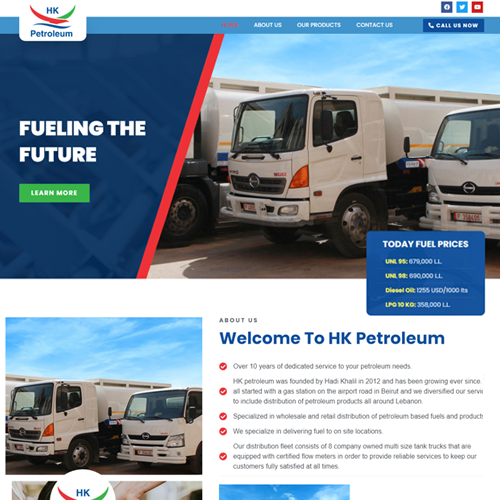This is a detailed description of an image showcasing the homepage of a website:

At the top of the homepage, a white navigation bar spans across the screen. On the left side of this bar, the website’s logo is displayed prominently. The logo consists of a white rectangle featuring the initials "HK" in blue font at the top, followed by a stylized bird design created from red swirls. Below this emblem, the word "Petroleum" is inscribed in blue font.

In the upper right corner of the white navigation bar, there are several social media icons that link to platforms such as Twitter, Facebook, and YouTube, allowing users to share content directly from the website.

Below the white navigation bar, a blue horizontal bar houses the website's main navigation menu. The menu is organized with options in red font, indicating that the current page is "Home." Other clickable options include "About Us," "Our Products," "Contact Us," and "Call Us Now."

The central portion of the homepage features a graphic representing three large, white tanker trucks that are typically used for transporting gasoline and oil. Adjacent to this graphic, on the left side, there is a red diagonal slash that separates it from a textured dark blue section. This section contains the tagline "Fueling the Future" in white font. Below this inspirational message, a red rectangle button with white font invites users to "Learn More."